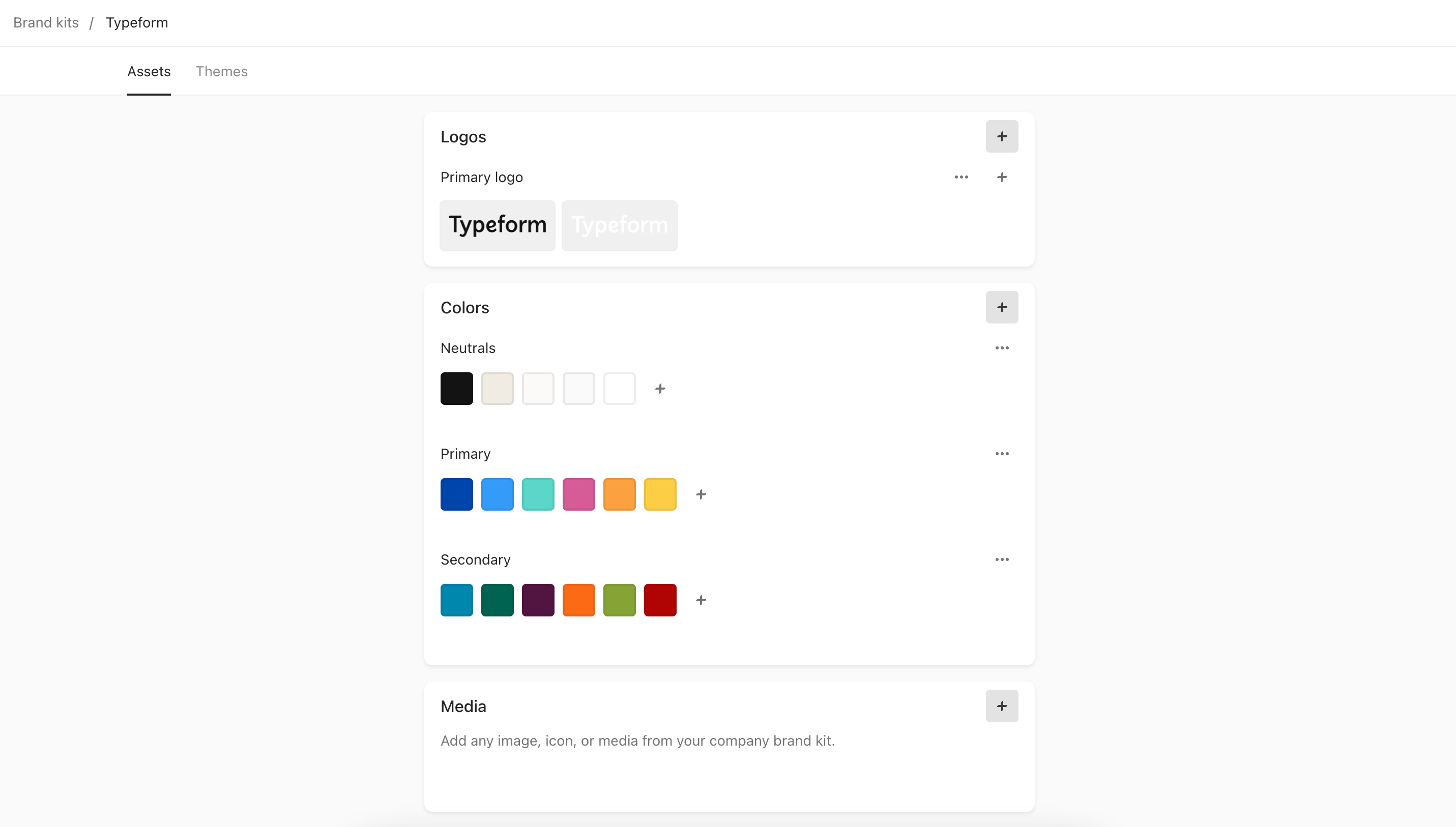Screen capture of a website's branding kit interface. The backdrop is white, with the top part featuring a header in a grayish-black font reading "Brand Kits / Typeform". Beneath this, a horizontal gray line spans the width of the page. Leaning towards the top-left corner, the label "Assets" is bolded in black with a black underline, and adjacent to it in gray is the word "Themes".

Centered on the page, three primary sections vertically align. The first, smaller in height, is labeled "Logos". Within it, two options for the primary logo are presented, both reading "Typeform". One resides in a gray box with bold black text, and the other in a gray box with bold white text. Each logo option includes a plus icon on the right for further actions.

The subsequent section, approximately two and a half times taller than the first, is categorized under "Colors". Subheading "Neutrals" sits atop five progressively lighter shaded boxes, ranging from black to pure white. Below, under the "Primary" heading, sit six color boxes displaying dark blue, light blue, seafoam green, pink, orange, and yellow hues. Following this, the "Secondary" section showcases another set of six color boxes: teal, green, purple, orange, lime green, and red.

The final section at the bottom, labeled "Media," provides space to add images, icons, or other media from the company's brand kit. Similar to previous sections, each box includes a plus icon at the top right, encased in a gray square, for uploading additional assets.